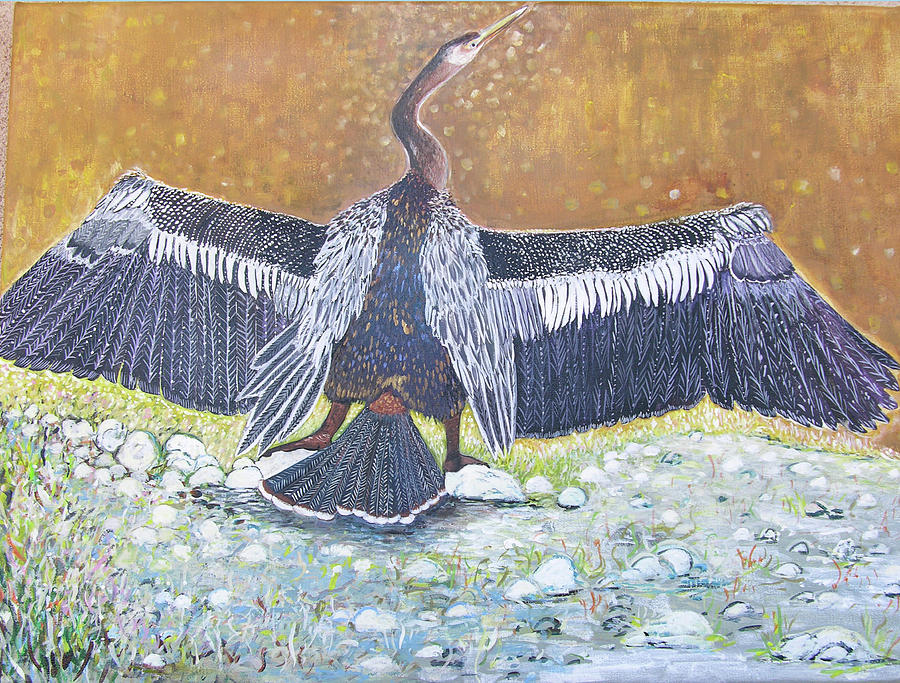This detailed painting captures a majestic, large bird with its back to the viewer, wings fully outstretched, presenting an awe-inspiring wingspan that spans nearly the entire canvas. The bird's long, dark reddish-brown neck arches gracefully, giving it a crane-like appearance, and transitions to a slender, pointed yellow beak. The eye area exhibits a slight white highlight, offering a sharp contrast. The bird's feathers display a spectrum ranging from dark navy blue on its back and wings, interspersed with white highlights and delicate patterns of black and blue towards the top edges. Its substantial tail feathers fan out in a triangular formation, marked with a gradient from a black base to white tips and edges of yellow. The legs and feet are distinctly reddish-brown and stand firmly on a terrain of white pebbly rocks, partially submerged in a flowing river, with some green grass patches emerging from the water. The background of the painting is a light brown hue, accentuated with touches of yellow, evoking a serene, natural environment. The intricate details of the feathers and the bird's poised stance exude an air of nobility, making this hand-drawn piece a striking representation of avian beauty.